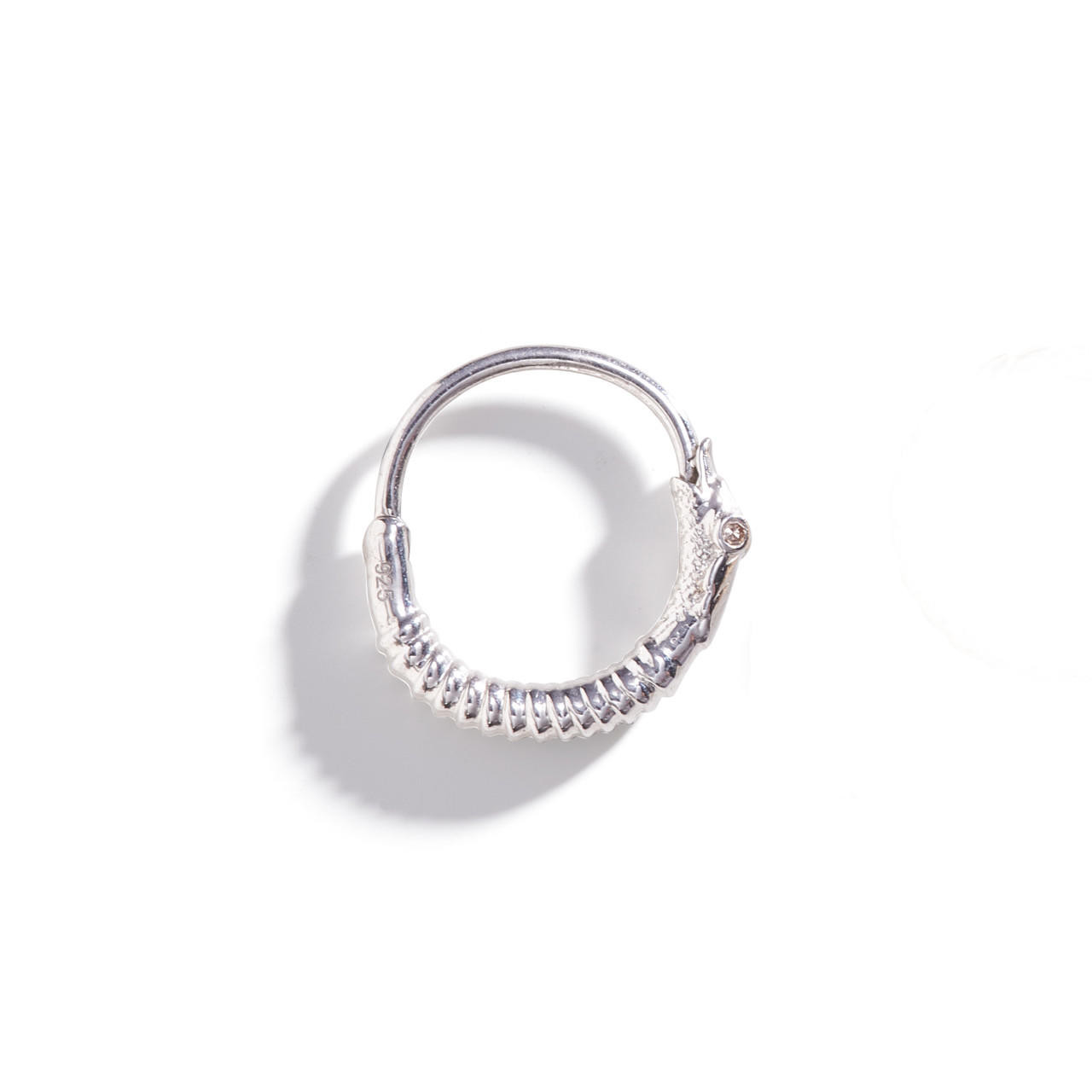The image depicts a single earring made of silver-colored metal, placed on a smooth white surface, likely a table. The earring, which has the shape of a small loop or a ring, shows varying textures; the top part is smooth while the bottom half is adorned with numerous bumps and grooves, giving it a detailed, almost caterpillar-like appearance. A distinct shadow is cast on the table by the earring, indicating a light source from above. On the left side of the earring, there is a set of engraved numbers, either "929" or "923," though the exact sequence is unclear. The overall design includes clip-on edges and exudes an intricate contrast between its smooth and textured sections.